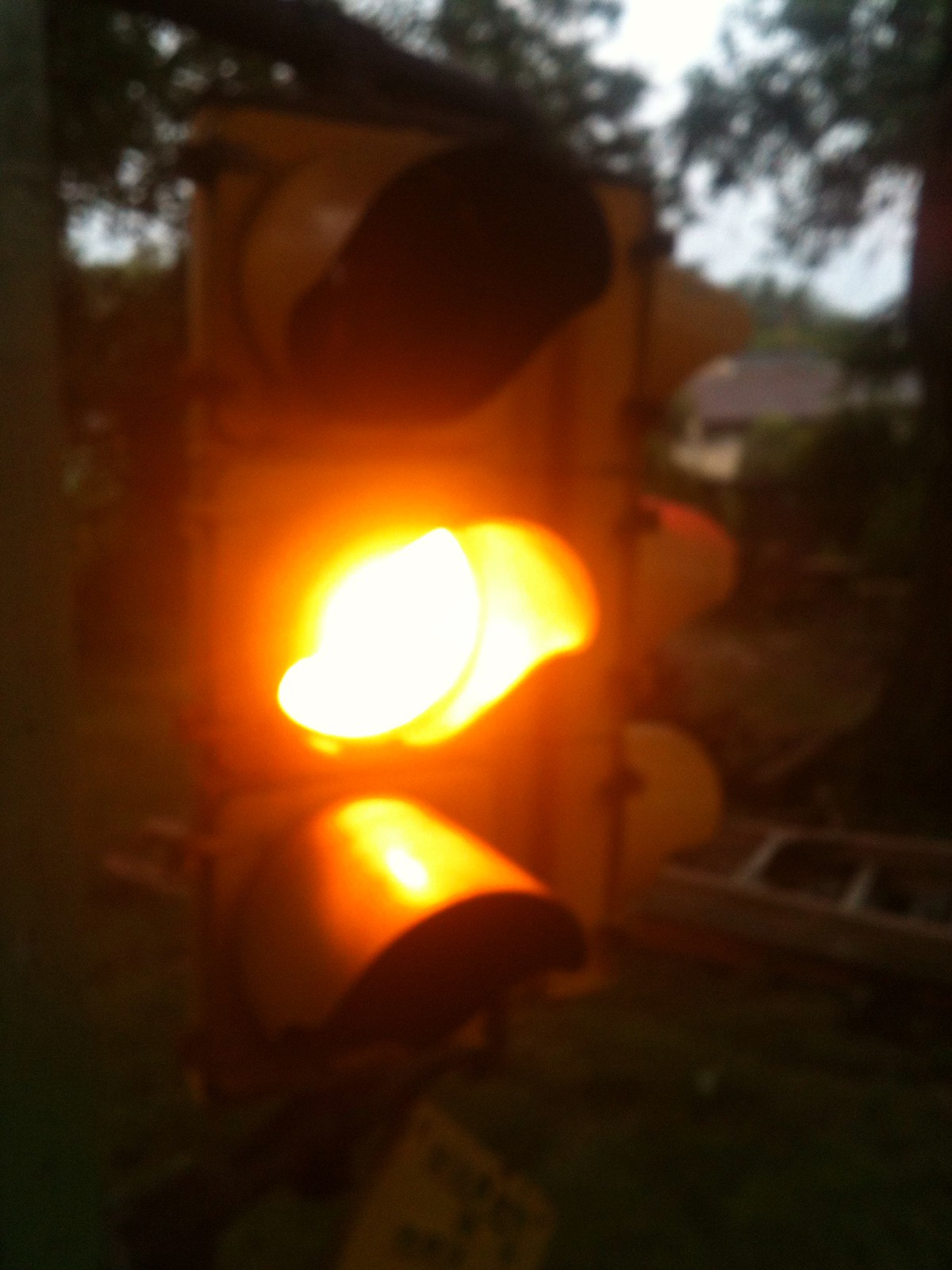A detailed scene unfolds in this photograph illuminated by a traffic signal. At the forefront stands a metallic traffic light, its yellow signal light glowing brightly beneath its distinctive hood. The structure displays three circular lights on its front, mirroring an identical arrangement on its right side.

Lying on the ground directly behind the traffic light is a ladder, stretching across the frame. Nestled underneath the ladder, a yellow sign adds to the complexity of the scene. To the back left and right, two trees rise, creating a natural archway that frames an opening between them.

In this opening, a dense hedge can be seen, adorned with a small, obscure white object. Farther in the background, peeking through the foliage, is the angular structure of a house roof, providing a subtle hint of suburban context to the otherwise urban foreground. The intricate details and layered elements in this shot weave a rich tapestry of visual interest.